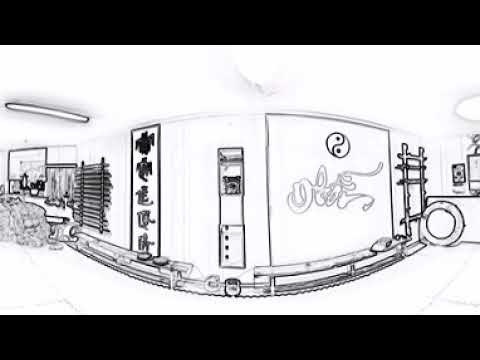The image is a detailed black and white line drawing of a living room-like space, presented in a convex rectangular layout that draws the viewer's eye inward. The room features numerous intriguing elements, including a swirling yin-yang symbol on the upper right side, although it deviates from the traditional design with neither a distinctly black nor white half. To its left, a vertical panel is adorned with what appears to be writing or symbols in a language other than English, evoking the feel of totems or ancient scripts. Below the yin-yang, there is a small structure resembling a shelf or ladder, bearing a round object similar to a life preserver. Additionally, the left side of the room showcases venetian blinds, while another poster hangs nearby, decorated with more complex designs that might depict dragons or mythical creatures. The ceiling is outfitted with contrasting light fixtures: an elongated oblong light on one end and a round light on the other, adding to the eclectic nature of the room’s décor.